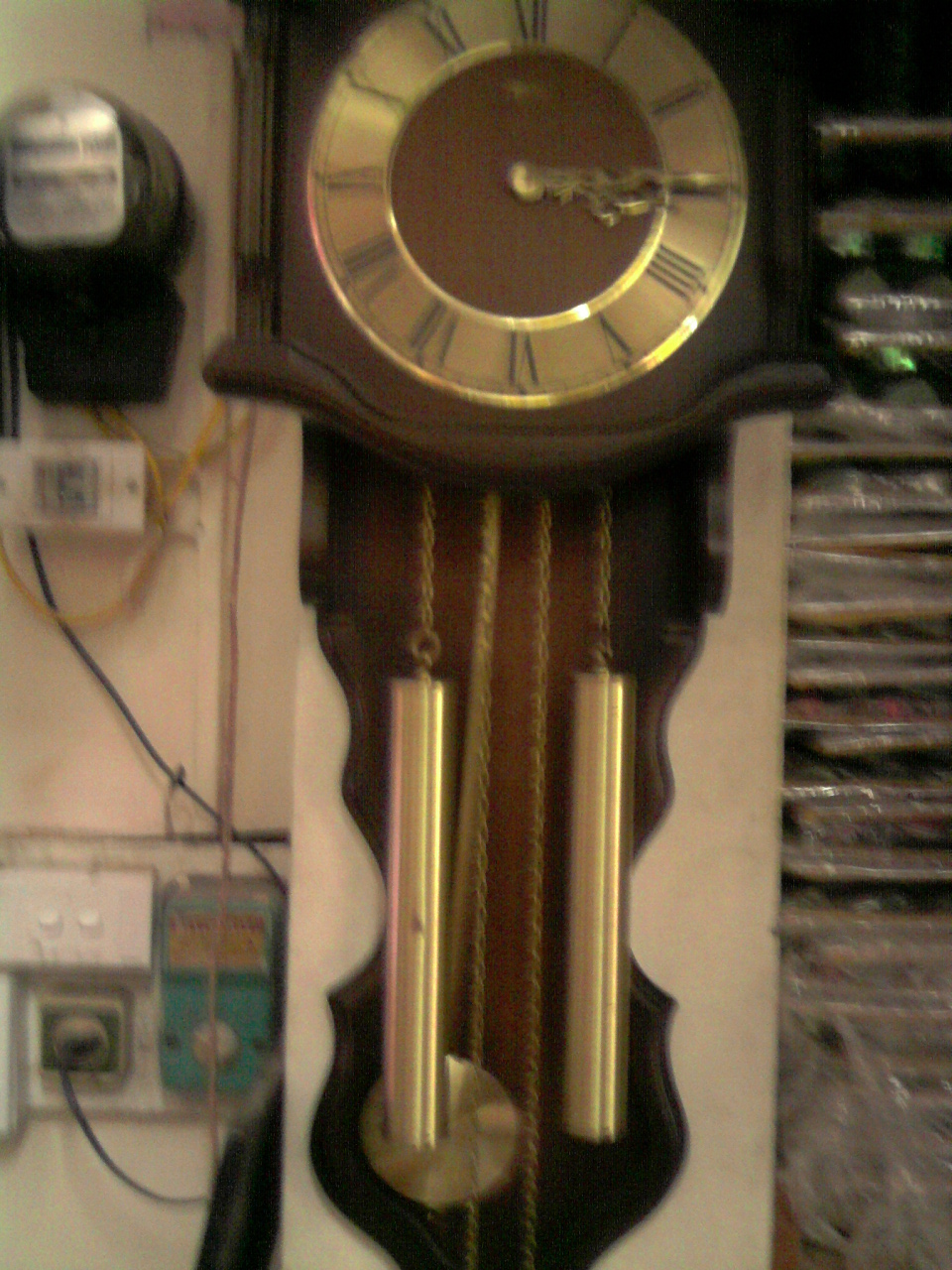The image features an old-fashioned grandfather clock with a richly detailed, dark wooden exterior accentuated by lighter wood carvings. The face of the clock, large and circular, is prominently gold and showcases Roman numerals. The hour and minute hands are also gold and are pointed towards the three. The clock includes intricate features such as golden poles and chains, which dangle from the body. A prominent golden circle can be seen hanging at the bottom. The clock, though slightly blurred in the image, hangs on a strip of drywall next to some wires, plugs, and other electronic equipment, contrasting its antique charm with the modern elements around it.